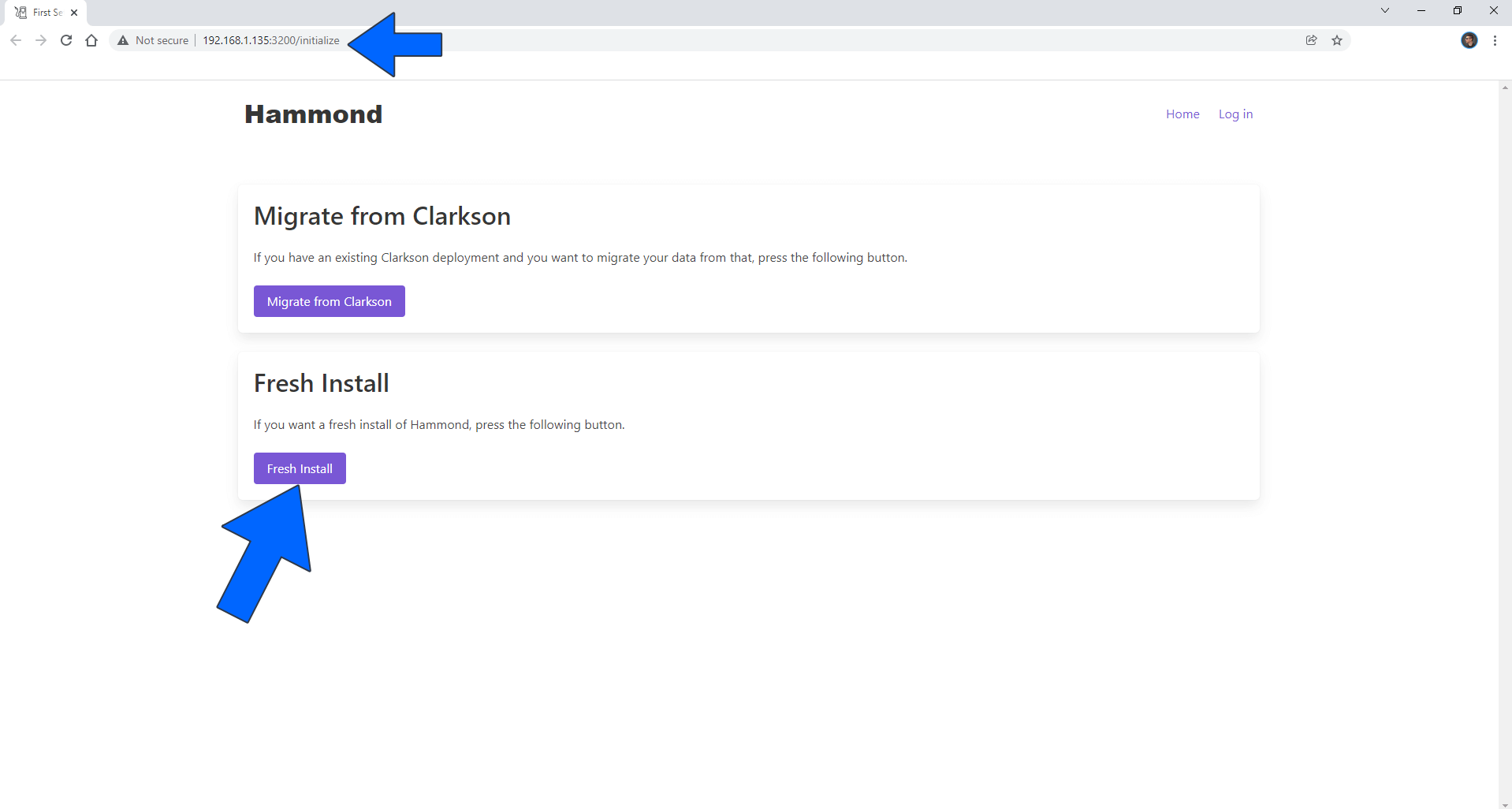The web browser is displaying a setup page for a router or network device. The address bar contains a local IP address, specifically "192.168.1.135:3200/initialize," indicating a setup phase for a device on the user's local network.

The webpage appears to be rather minimalist, with "Hammond" indicated at the top—though "Hammond" isn't a commonly known router brand. On the top right corner, there are navigation links labeled "Home" and "Login."

The main content of the page consists of two prominent white boxes with gray shadows to highlight them. The first box, titled "Migrate from Clarkson," provides an option for users to migrate data from an existing Clarkson deployment, accompanied by a button labeled "Migrate from Clarkson." The second box, labeled "Fresh Install," offers the option to perform a fresh install of the Hammond system, with a corresponding button labeled "Fresh Install." 

The page serves to guide the user through either migrating from an existing setup or initializing a new setup for the device.